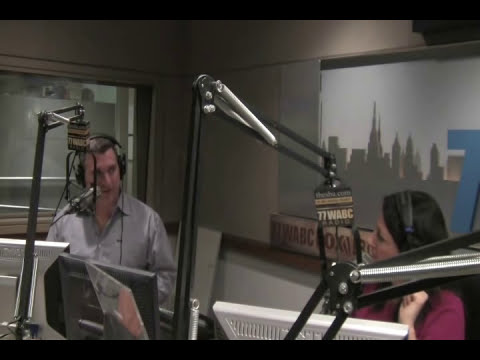In this detailed full-color photograph, a radio station studio is depicted, framed by thin black borders on the top and bottom, and oriented horizontally. The scene captures the intersection of two studio walls: the left wall features a large plate glass window, and the right wall displays a faux cityscape background adorned with the "W.A.B.C." logo. Central to the image are two individuals—a man and a woman—sitting at computers spaced approximately six feet apart. Both are equipped with headsets and are speaking into large mic booms labeled "77WABC," indicating their role as radio hosts or guests on the New York-based station. The woman, positioned on the right, wears a purple-pink shirt, while the man on the left is clad in a light blue, partially unbuttoned, button-up collared dress shirt. The studio is filled with multiple computer monitors, with some white and some black, adding to the professional ambiance of the recording environment.